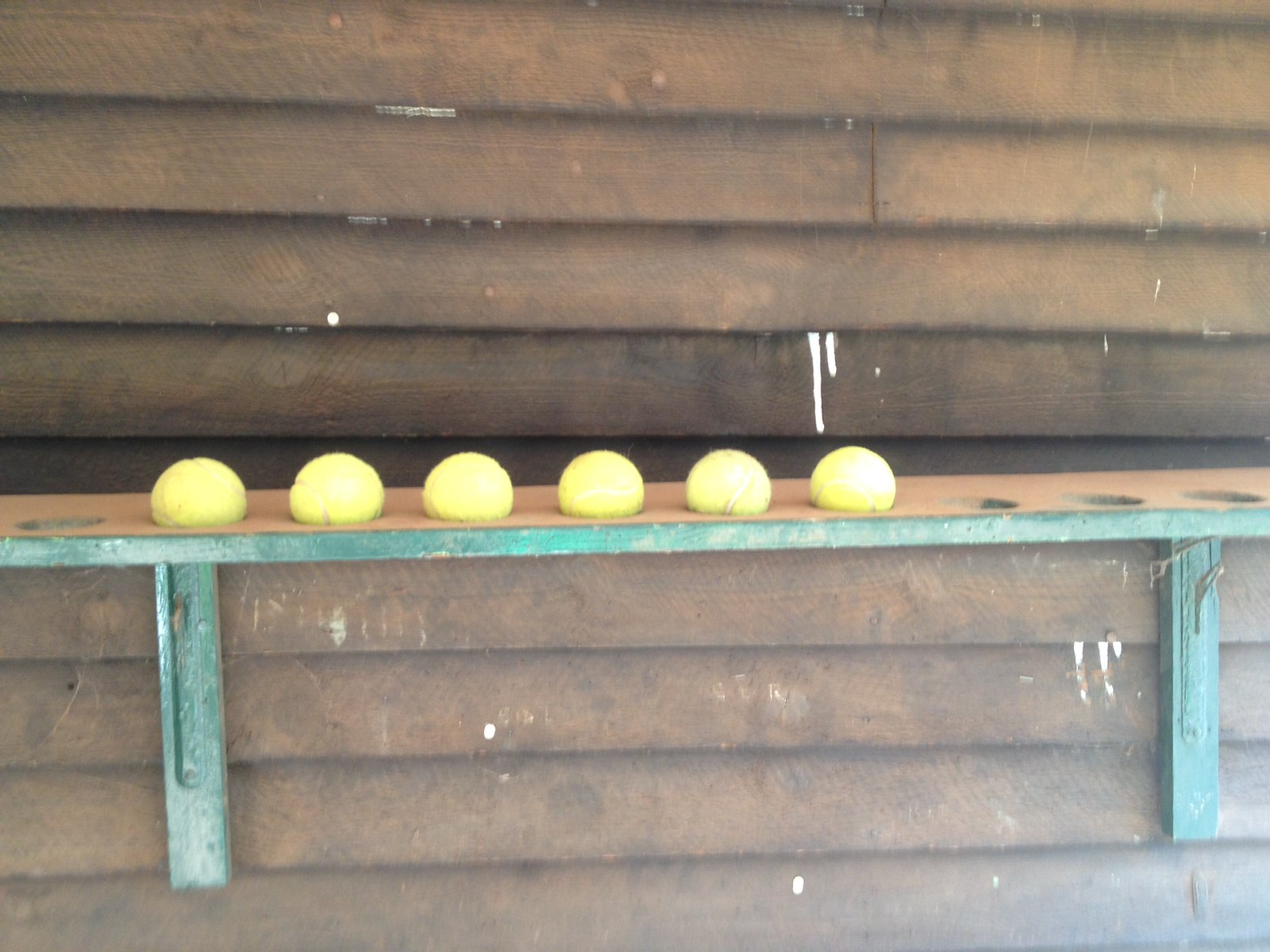The image features a detailed scene of a rustic, brown wooden wall with a clapboard design, characterized by overlapping wood planks and occasional drips of white paint. Affixed to this wall with green-painted brackets is a specially designed wooden shelf, which is partially painted green. The shelf itself holds six neon yellow tennis balls, each perfectly placed in circular cutouts designed to cradle them. The shelf extends horizontally across the center of the image, displaying its simple yet functional design. Despite its utilitarian purpose, there's a touch of neglect shown by noticeable cobwebs on the underside and dust on the top. Overall, the image captures a harmonious blend of utility and rustic charm.